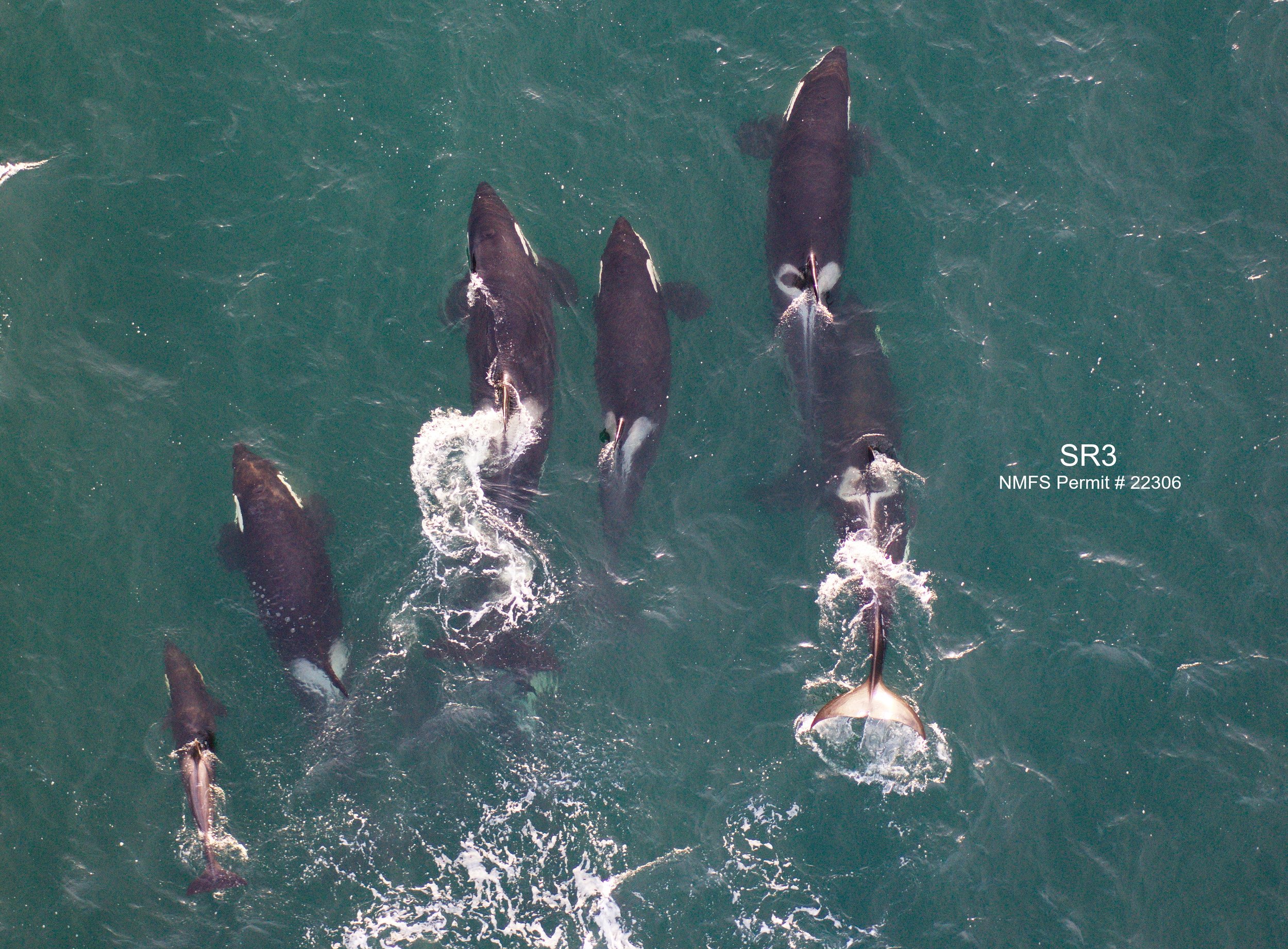This aerial drone photograph captures a pod of six killer whales, also known as orcas, swimming in a body of deep teal water. The image, taken straight from above in a landscape orientation, shows the majestic orcas in various stages of movement. The whales' black, sleek bodies and distinctive white markings on their fins and cheeks are visible from this high vantage point. Among the pod, most appear to be adults, with at least one juvenile whale noticeable in the lower left part of the frame. The whales are leaving foamy trails in the slightly wavy water as they swim towards the upper side of the image, with one whale prominently showing the white of its tail above the water. On the right side of the image, white text reads "SR3 NMFS permit number 22306."